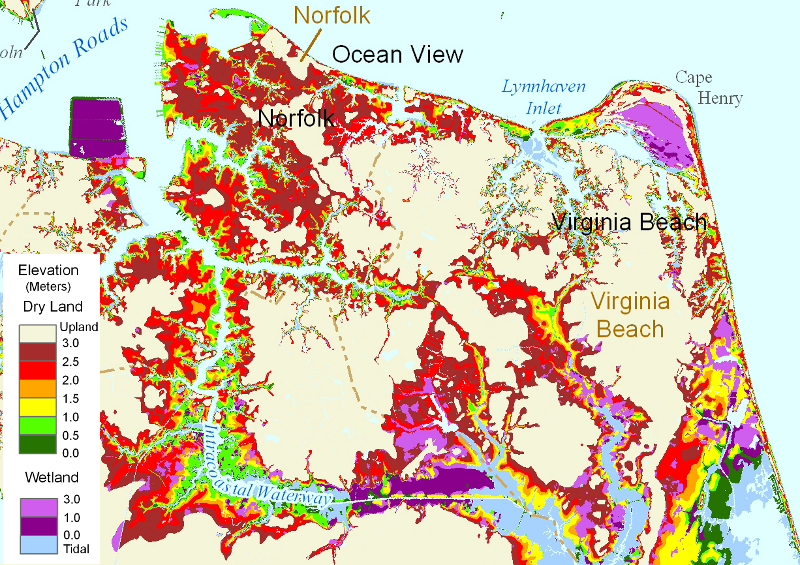This image is a detailed scientific map depicting the elevation and land classification of the Virginia Beach area, including Norfolk, Ocean View, Cape Henry, and surrounding regions. The rectangular landscape map shows various elevation levels measured in meters, using a color-coded system for clarity. Dry land is indicated by shades ranging from light gray and green to dark red, with the most common color being a tannish-beige, representing higher upland areas. Wetlands are shown using light blue, lavender, and darker purple hues, indicating lower-lying, tidally influenced regions. The map features notable landmarks such as the Intracoastal Waterway, Hampton Roads, and Lynnhaven Inlet, with elevation variations largely corresponding to proximity to the ocean and rivers. A key in the lower-left corner provides a guide to the colors, showing values from 0.0 to 3.0+ meters for both dry and wet lands. Labels, in both black and tan brown, highlight significant areas, and color gradients delineate the transition from high upland regions to lower wetlands, effectively illustrating the varying elevation and land types across this coastal portion of Virginia.